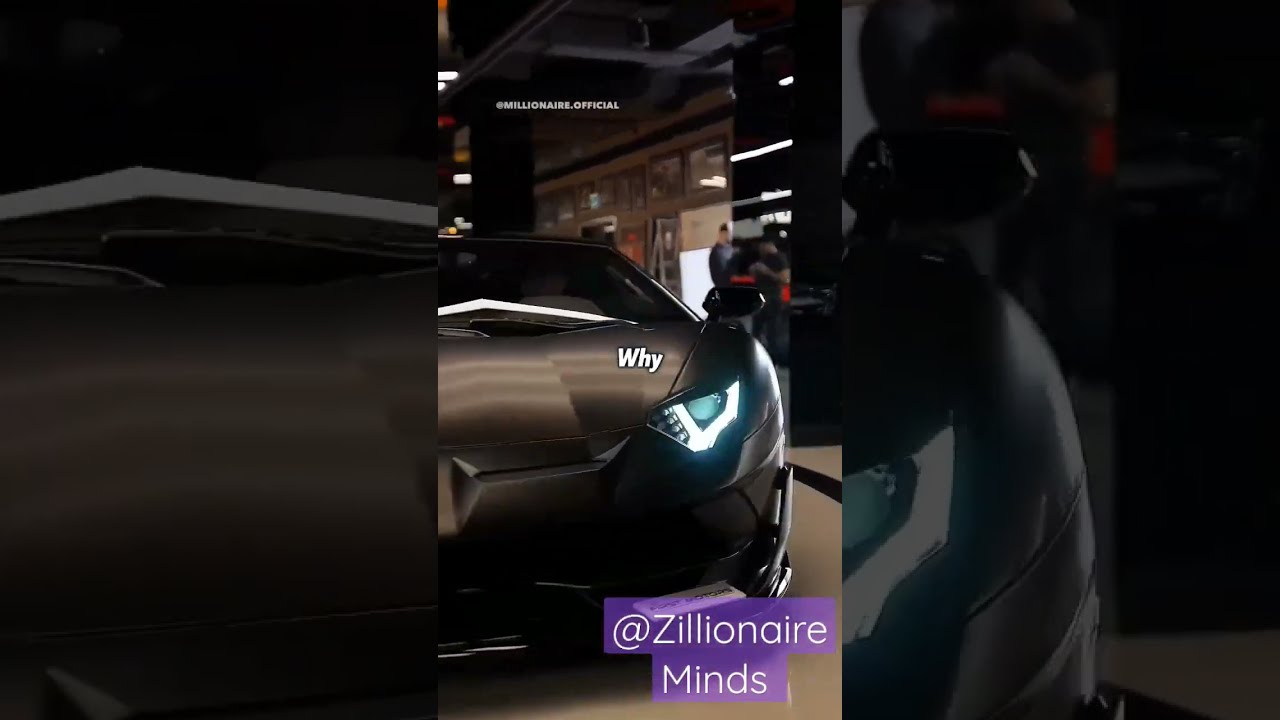The image depicts a scene inside an auto body shop or a mechanics place. The overall ambiance is quite dark, making it somewhat challenging to discern the details clearly. The focal point is the front end of a car, which is painted in a metallic brown-gray shade. The car features a striking blue headlight that resembles an eye. Dominating the hood of the car is the word "WHY" written in capital white letters. 

The picture seems to be divided into thirds, with the left and right sections featuring darker, enlarged, and obscured images of what appears to be the same car, adding a sense of mystery to the composition. In the top part of the photo, there is small white text that reads "@millionaire.official," while the lower right corner features a highlighted purple section with white text that says "@zillionaire.mines." 

In the background, you can spot people working, reinforcing the auto shop setting and adding to the dynamic atmosphere of the image.